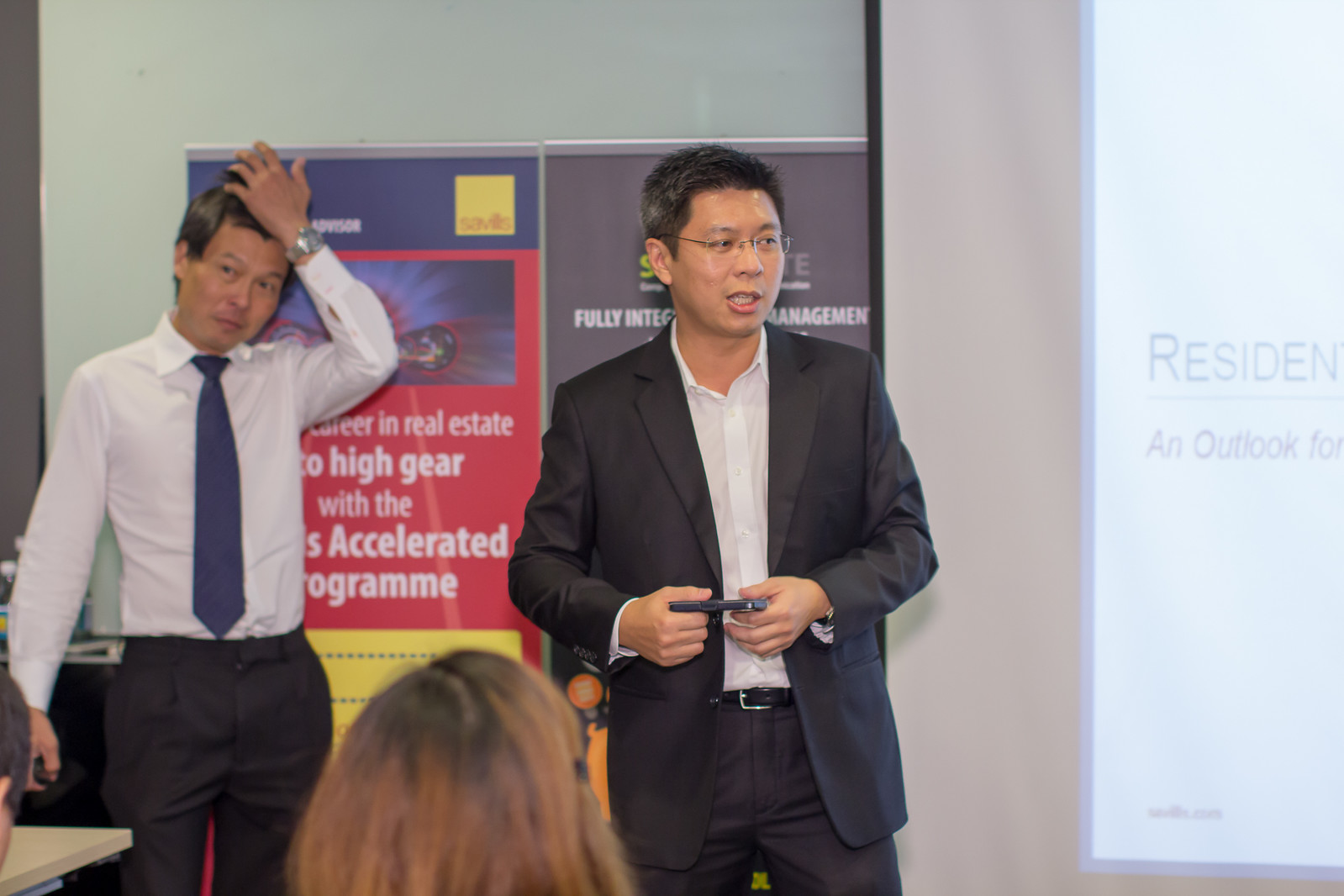In this image, two men, appearing to be Asian, are positioned at the front of a light-blue, well-lit room, seemingly involved in a presentation. The man in the foreground, likely the main speaker, is dressed in a dark gray or black suit with a white button-up shirt that is open at the collar. He wears rimless glasses and holds a device, possibly controlling slides or visuals. His short black hair is interspersed with gray, and his attention is directed off to the side.

Standing slightly behind and to the left of the speaker is another man, dressed in a white button-up shirt and blue tie, with his shirt tucked into black or gray pants. This man sports a silver watch on his left wrist and is scratching his head with his left hand, suggesting a moment of frustration or contemplation. His black hair and absence of a jacket give a casual yet professional appearance.

Behind them, there is a red sign with white lettering about careers in real estate, specifically mentioning an "accelerated program" and "high gear." Adjacent is a gray sign whose details are obscured. A projector screen displaying the word "resident" is partially visible to the right, hinting at an ongoing slideshow or presentation. In the audience, only the back of one person's blonde head is visible, suggesting more attendees out of the frame. A desk in front of the speaker also indicates a formal setting, likely a seminar or business meeting room.